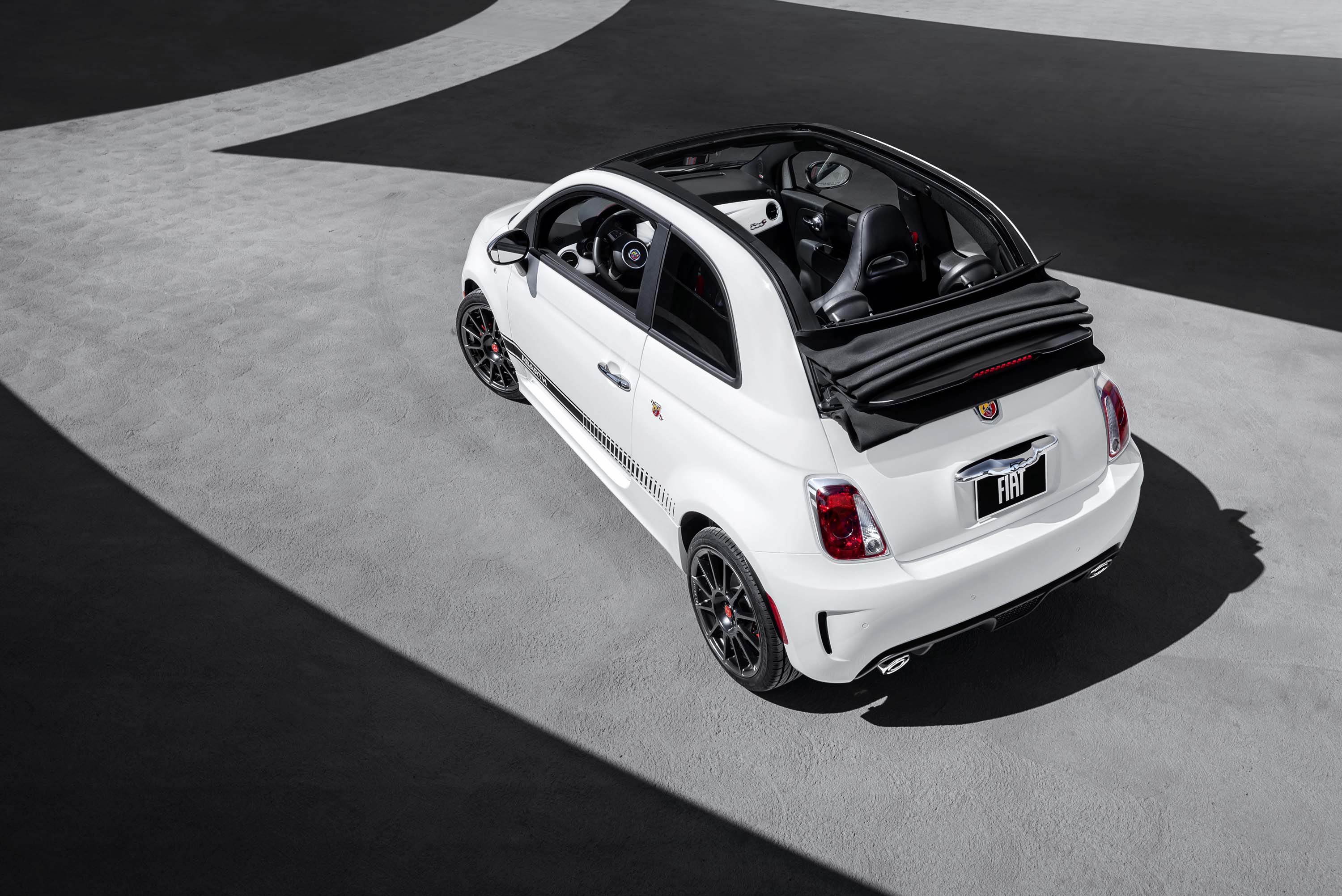The image depicts a compact, all-white Fiat convertible parked on a gray, patterned road surface. The cement ground beneath the car features a distinct wide white band resembling the letter "M" and other narrow bands, adding depth to the scene. The Fiat sits slightly diagonally to the bands, showcasing its design details. Notably, it has its black retractable roof down, clearly presenting the black interior and contrasting white dashboard. The exterior is enhanced by black tires with red centers, black-rimmed rims, and a decorative line along the side that transitions from solid to dotted black. The back of the car displays a Fiat license plate with white text on a black background, as well as rear lights that are white and red. A yellow and red emblem and silver door handles add finer detailing to this stylish vehicle, which sits in a setting that blurs the lines between an outdoor and showroom environment.